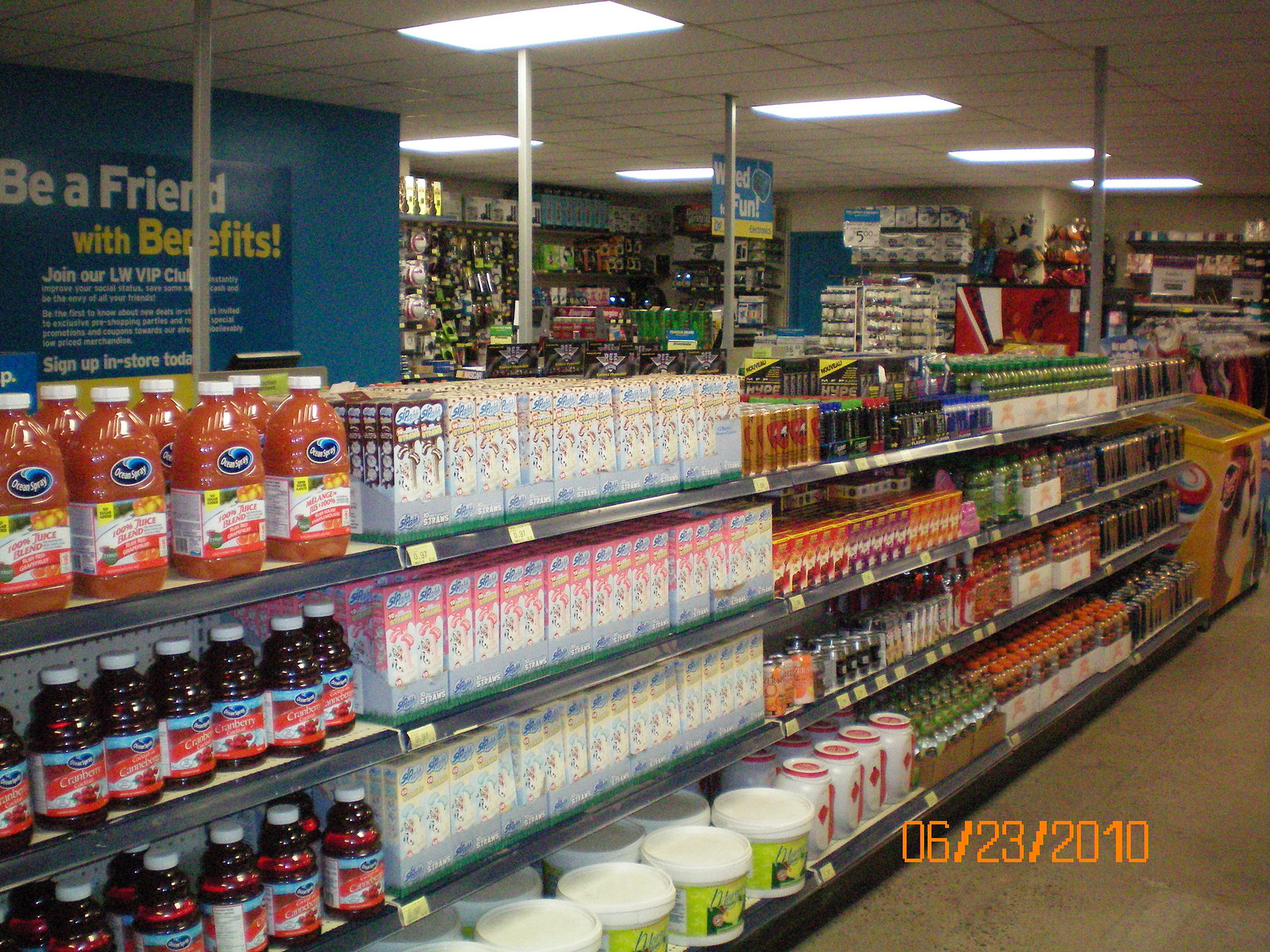The image depicts a quaint, rustic store reminiscent of a camping supply shop. The interior features aging ceiling paneling, reminiscent of cork, with simple lighting fixtures illuminating the space. The shelves are stocked with various items, including Ocean Spray juices and an assortment of sodas. Toward the end of the aisle, there is an ice cream freezer with a selection of frozen treats. In the background, a small round rack displays clothing, and there is possibly a stand for sunglasses. The store has a charming, multi-purpose appeal, offering a variety of goods from beverages to apparel.